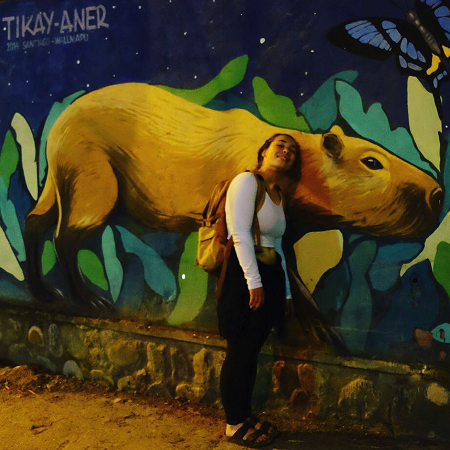The photograph showcases a young woman leaning against a mural on an outdoor stone wall. The mural depicts a large brown capybara under a night sky filled with stars and a butterfly or moth in the top right corner. Surrounding the capybara is lush greenery in varying shades of light and dark green, casting shadows that add depth to the image. The woman, donned in a white long-sleeved midriff blouse, black yoga pants, sandals, and carrying a yellow backpack, is positioned towards the capybara's head, her head tilted as she gazes directly at the camera. The stone wall beneath the mural is embedded with various stones, and the ground below is a tightly packed dirt road. At the top-left corner of the mural, partially obscured text reads "T-I-K-E-Y dash A-N-E-R."